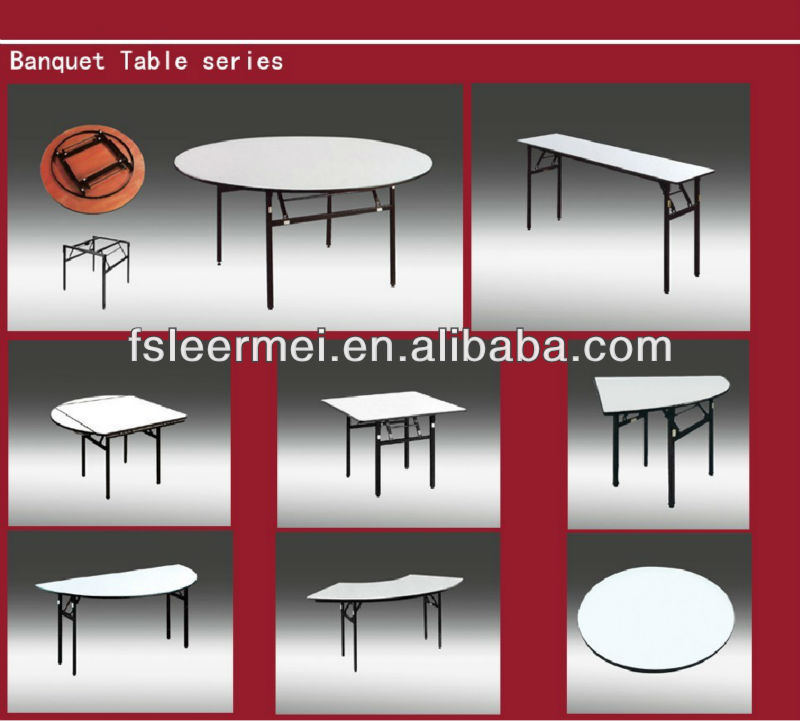The image is a square, product-centric promotional graphic typically found on a manufacturer's site. The background is a solid red gradient with multiple digitally-created table images arranged in three rows: two images on the top row, three in the middle, and three on the bottom. At the very top, a white horizontal line spans the width of the image, beneath which the title "Banquet Table Series" is prominently displayed in white text.

The top row features a versatile round table on the left, depicted in three stages: fully assembled, the tabletop flipped upside down, and the base alone. To its right is a tall, rectangular table. The middle row starts with a modular table that can be either square or round, followed by a square table in the center, and a quarter-moon-shaped table to the right. The bottom row includes a half-moon-shaped table on the left, a curved desk-like table in the middle, and concludes with a solid round tabletop on the far right.

At the very center of the graphic, the URL "fsleerm-ei.en.alibaba.com" is displayed, suggesting a direct link to the product's page. The detailed, computer-generated images and clean organization emphasize the variety and adaptability of the banquet tables available.